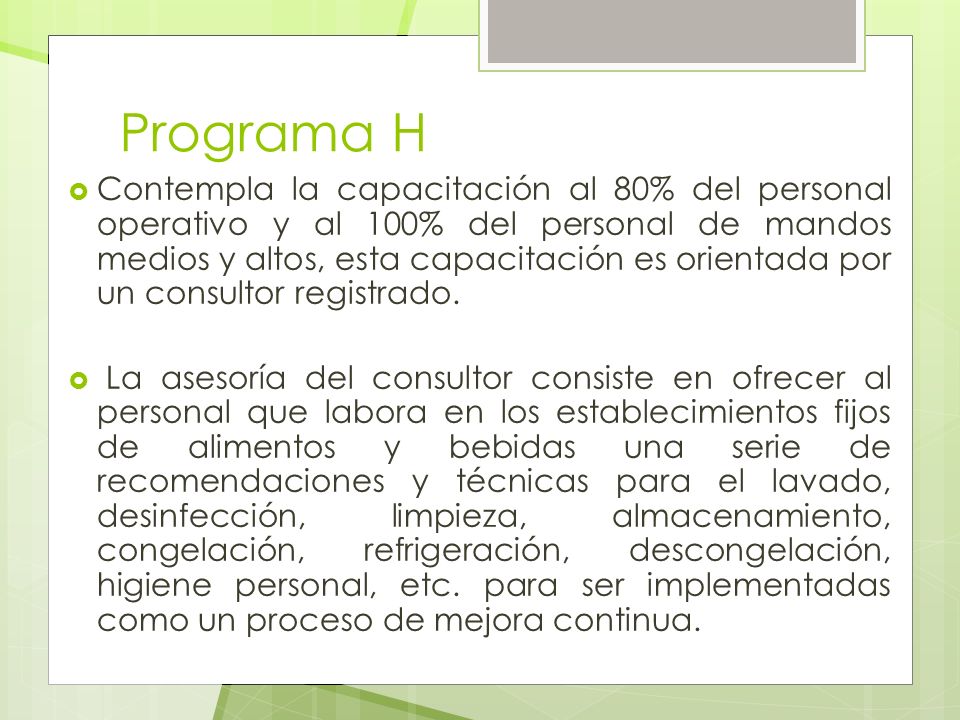This image features an informational poster, predominantly in Spanish, with a clean and structured design ideal for a PowerPoint presentation. The poster is framed with a grayish-green border, adding a professional touch to the overall aesthetic. Inside, a white background provides a clean slate for the text, which appears to be centrally aligned.

At the top of the poster, the heading reads "Programa H" in light green text. Below the heading, the body of the poster contains two bullet points, each marked by hollow green circles. The first bullet point, written in blue text, states "Contempla la capacitación al 80% del personal operativo y al 100% del personal de mandos medios y altos. Esta capacitación está obteniendo por un costuletar registrado." The second bullet point, larger in size and black in color, features additional details in Spanish. The design elements include a light green rectangle with lines and a cut-off dark gray square, positioned at the top left or right portion of the frame, adding visual interest to the poster.